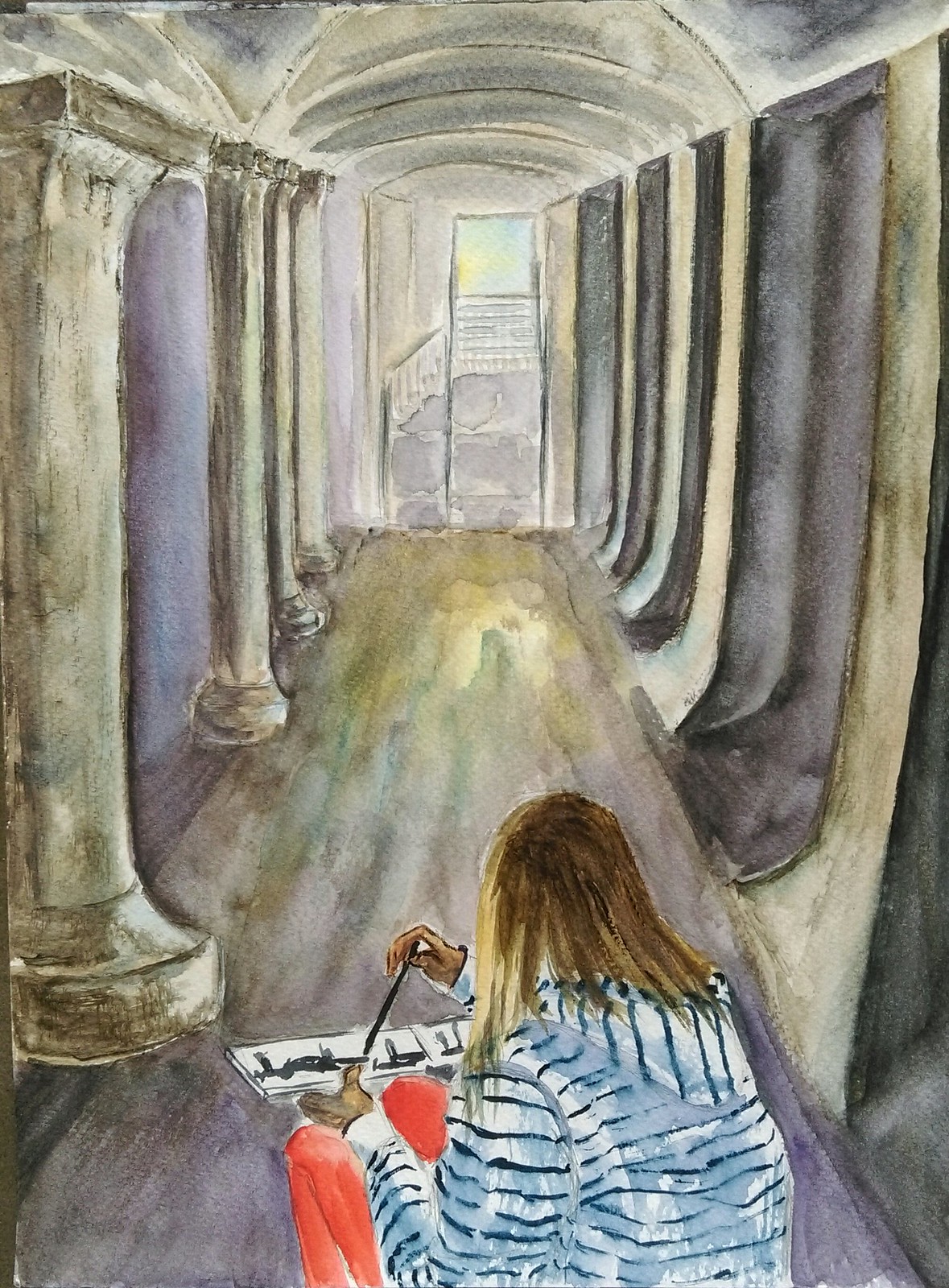The image is a detailed watercolor painting of a long, arched ceiling hallway with distinct architectural features. On the left side, white pillars stand prominently, growing larger towards the bottom of the picture, and are complemented by a bluish-gray wall. The right side features more minimalistic, curved pillars with dug-out trenches in the wall. 

The hall leads to an open doorway at the end, where a glimpse of a yellow-green sky can be seen. The doorway itself is on the left of the center, marked by a small window and opening onto a staircase leading outward. The sunlight from above casts a yellow glow on the floor, transitioning to a duller gray closer to the foreground.

In the center foreground, a young woman with long, brownish hair streaked with blonde at the front sits on the floor with her back to the viewer. She is engrossed in her art, wearing red or orange pants and a white hoodie with thin blue or black stripes. Her left hand holds a palette with various colors, while her right hand wields a black paintbrush or pen, suggestive of intricate drawing or calligraphy. She sits partly crouched, seemingly lost in thought as she creates her artwork.